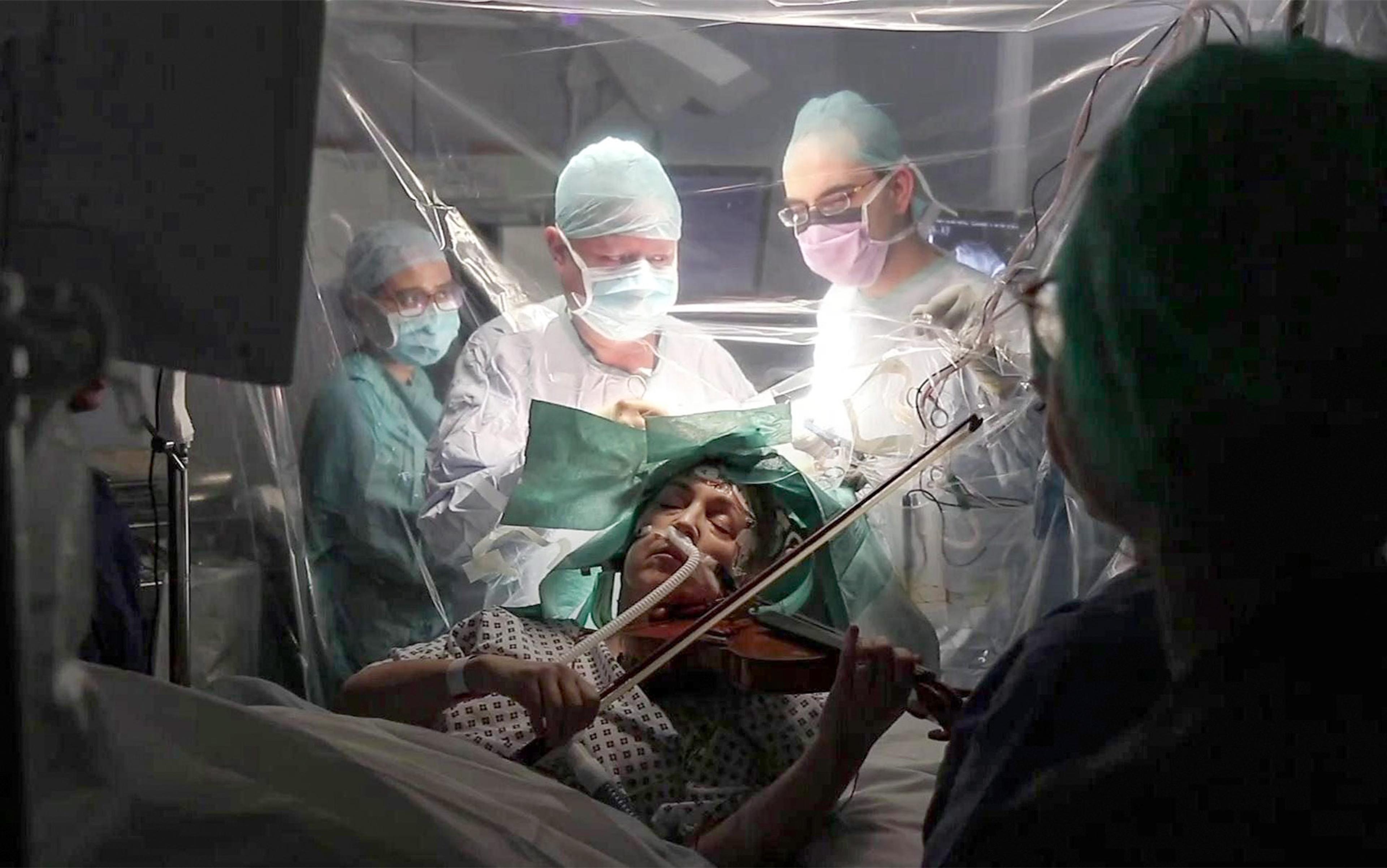In the operating room, a team of surgeons performs a complex brain surgery on a woman. Remarkably, the patient is seen playing the violin, with a bow held in her right hand and her eyes serenely closed, despite the delicate procedure. She is lying down under a sheet, her head surrounded by surgical paper, indicating the sterile environment. A bright surgical light illuminates her head, ensuring precision for the medical team. The woman is wearing a hospital gown and appears to be on oxygen, which is likely aiding her breathing during the operation. Two male surgeons, one carefully handling surgical instruments and the other in eyeglasses focusing intently on the procedure, are positioned behind her. In the background, a woman in surgical attire and another individual whose silhouette is only partially visible, also wearing glasses, appear to be assisting or observing. Surrounding equipment and plastic coverings add to the clinical atmosphere of the room. The juxtaposition of the patient’s musical performance and the life-saving surgical intervention highlights the extraordinary blend of medicine and artistry being employed.